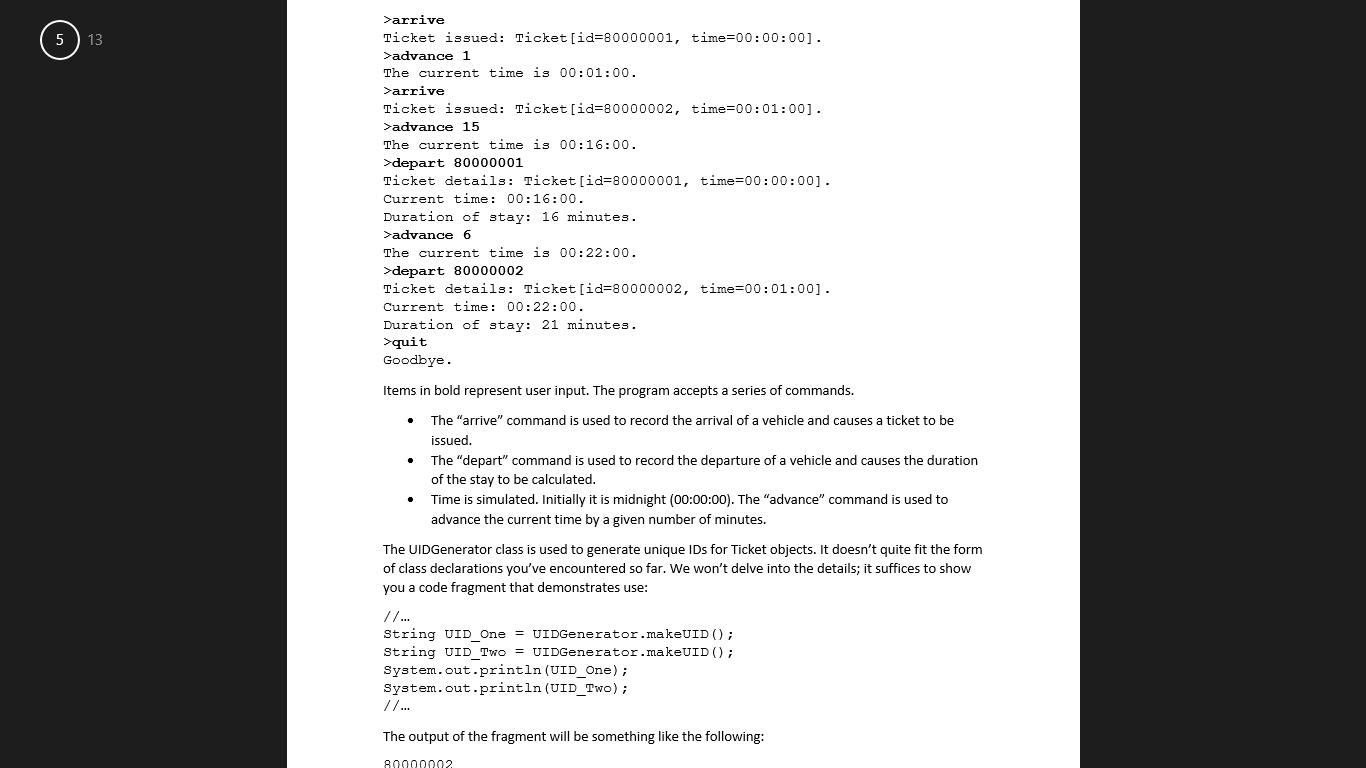**Detailed Caption:**

A web page provides real-time tracking information for vehicle tickets using a structured interface with commands represented in bold and capitalized text. The process starts with the **ARRIVE** command, which records a vehicle's arrival, logs the current time, and issues a ticket. For instance, at 1:00, the page shows "**ARRIVE**" followed by "TICKET ISSUED, TICKET ID, TIME ADVANCE 1." The **DEPART** command is used similarly to log the departure time and calculates the duration of the stay. At 16:00, a "**DEPART**" command logs that a vehicle departed, stating "TICKET DETAILS, TICKET TIME, CURRENT TIME 16:00, DURATION OF STAY 16 minutes," indicating the total time the vehicle stayed. Additionally, to simulate the passage of time, the **ADVANCE** command is used. For example, "**ADVANCE 6**" moves the current time forward by six minutes, showcasing a timestamp reading 22:00 with a corresponding departure command "**DEPART 800002**," alongside "TICKET DETAILS, TICKET TIME, CURRENT TIME 22:00, DURATION OF STAY 21 minutes." The interface concludes operations with the "**QUIT, GOODBYE**" command. This system utilizes a unique ID generator class to produce distinct ticket IDs, ensuring each ticket is individually identifiable. The output generator would produce results similar to the described scenario, effectively demonstrating the system's functionality.